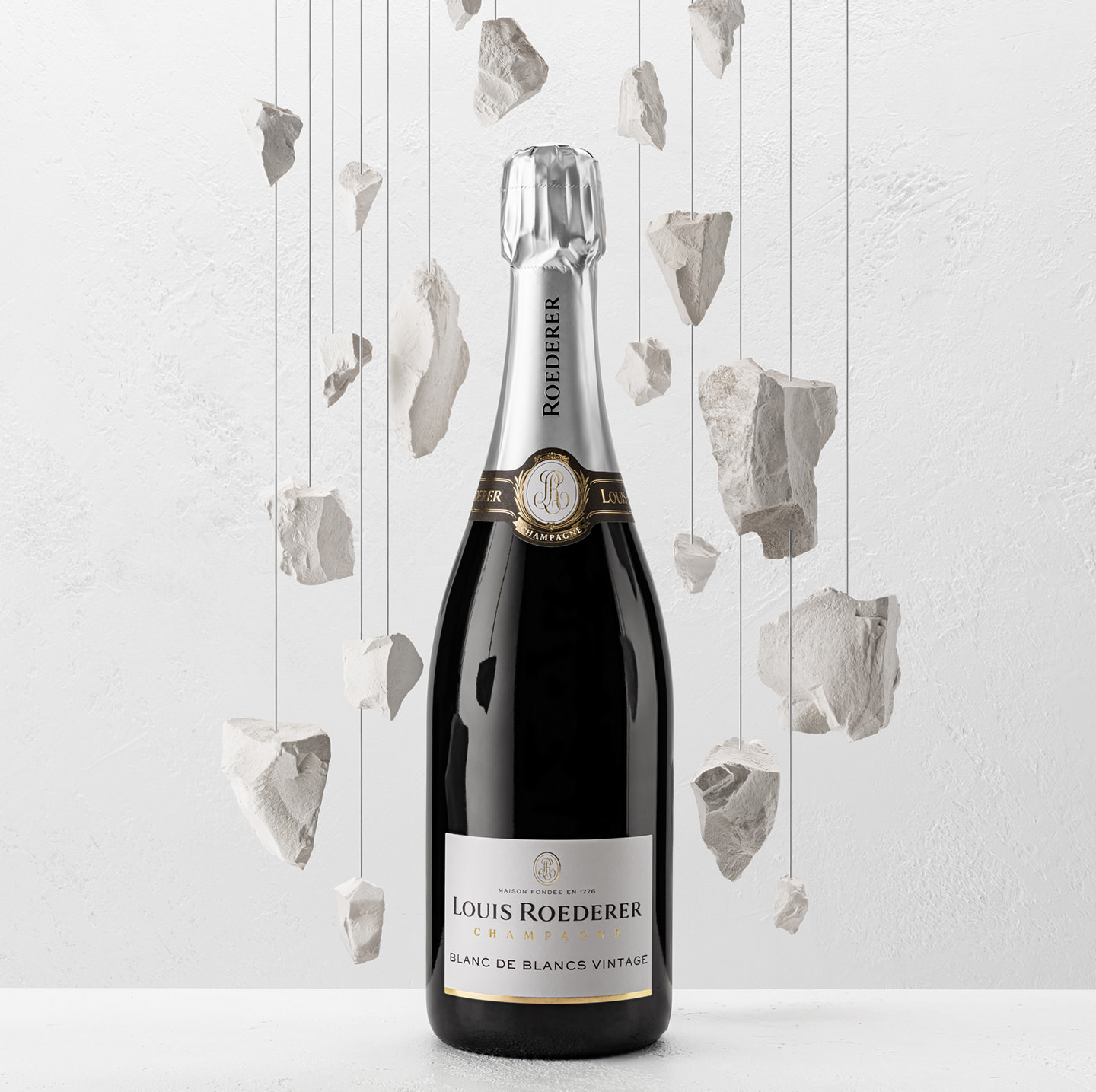This is a detailed photograph of a black bottle of Louis Roederer Champagne, specifically the Blanc de Blancs Vintage. The bottle features silver wrapping at the top, emblazoned with a crest emblem featuring the letter 'R'. The primary label underneath reads "Maison Fondé en 1776, Louis Roederer Champagne Blanc de Blancs Vintage," set against a brown and gold background with a white emblem. The bottle sits on a white countertop. The backdrop of the image is a white, textured wall with strings or wires hanging from the ceiling. Suspended from these strings are numerous white, beige rocks, possibly made from marble or concrete. This unique setup adds an interesting visual element to the composition, giving it an avant-garde advertising feel.